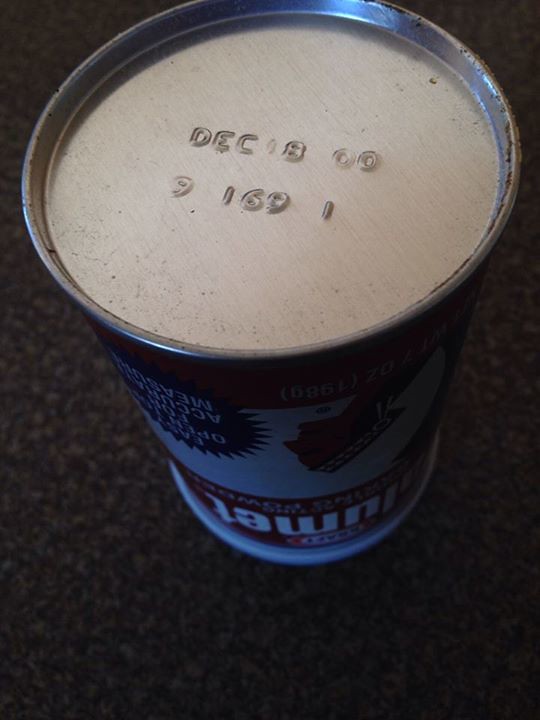This is an indoor photograph of an aluminum can, positioned upside down on what appears to be a kitchen counter with a dark, marbled surface featuring light brown speckles. The can's bottom is prominently displayed in the upper half of the image, showing its silver metal base. Indented into this base is the use-by date "December 18, 00" alongside a batch number "91691". The can itself has a label that is difficult to read due to the angle and lighting, but it seems to be predominantly dark red with a white band and white lettering. There is also an image of a person on the side of the can. The overall lighting of the photograph is quite dim, making it challenging to discern additional details on the can's label.